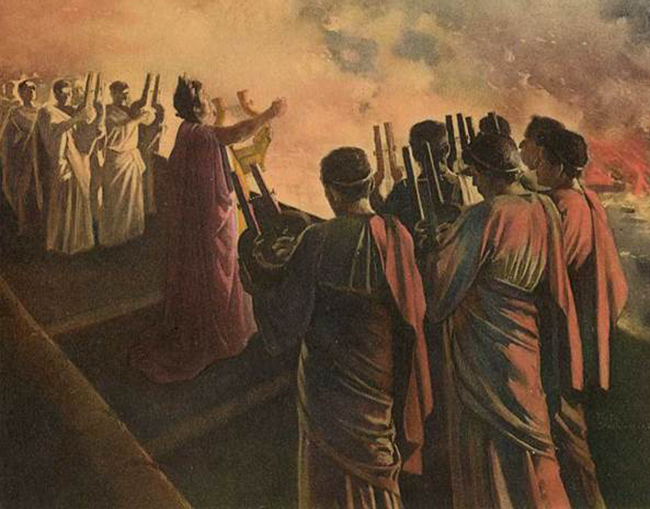The painting depicts a dramatic scene that appears to take place on a high wall or embattlement. To the left, five individuals clad in white robes hold sticks, while on the right, six individuals in red robes with gold embroidery hold similar sticks. The focal point is a central figure in a uniquely colored robe and a pink crown, holding up a golden object. This central figure is a female, and she gazes skyward with one arm extended, possibly invoking a biblical or historical context. The background reveals a burning city on the far right, with vivid orange and red flames and billowing white and gray smoke. The overall color palette appears faded, suggesting the painting's great age. All figures seem engaged in the scene, standing on the high structure, contributing to the dramatic tension as they observe the conflagration below.